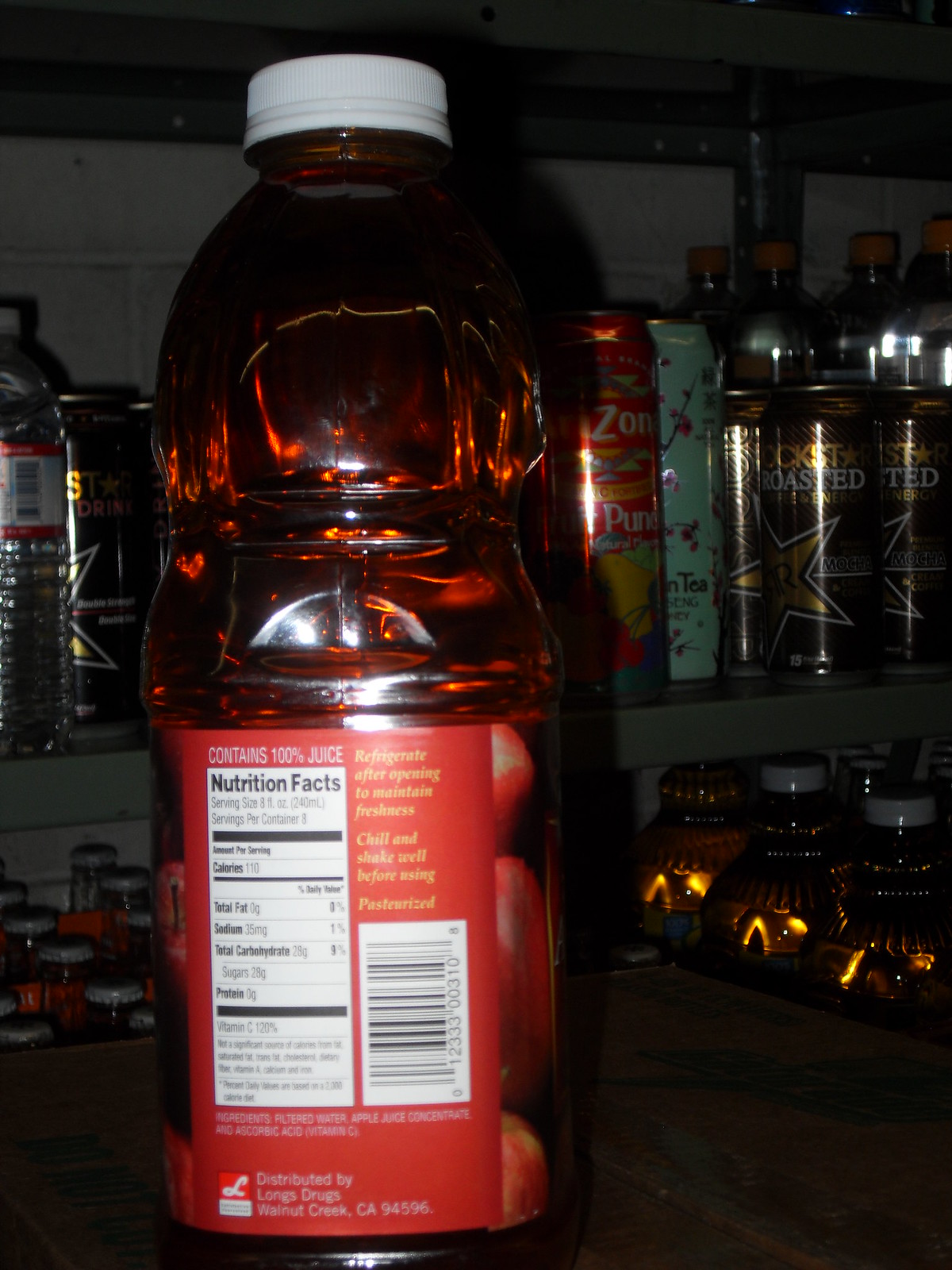The image captures a bustling kitchen scene centered around a large, clear bottle of red juice with a white cap. The red juice likely contains apple and cranberry, inferred from the label details which indicate it is made with filtered water, apple juice, and other ingredients. The label is a striking red, adorned with white text that includes "contains 100% juice" and a creamy detail of the nutrition facts indicating 110 calories per 8-ounce serving, with a total of eight servings in the bottle. Additional elements on the label like “pasteurized" and storage instructions like "refrigerate after opening" are visible but slightly blurry. A barcode is oriented vertically on the side of the bottle.

The bottle sits prominently on a wooden countertop, surrounded by a varied assortment of drinks in the background. Among these are glass bottles of juice with white caps, an Arizona iced tea can, a Rockstar energy drink, bottled water, and what appears to be Stewart's iced tea. The backdrop includes a white kitchen wall, hinting at this being a storage shelf or beverage area. The meticulous description of the scene provides a rich context, enhancing the visual depiction of this everyday kitchen moment.